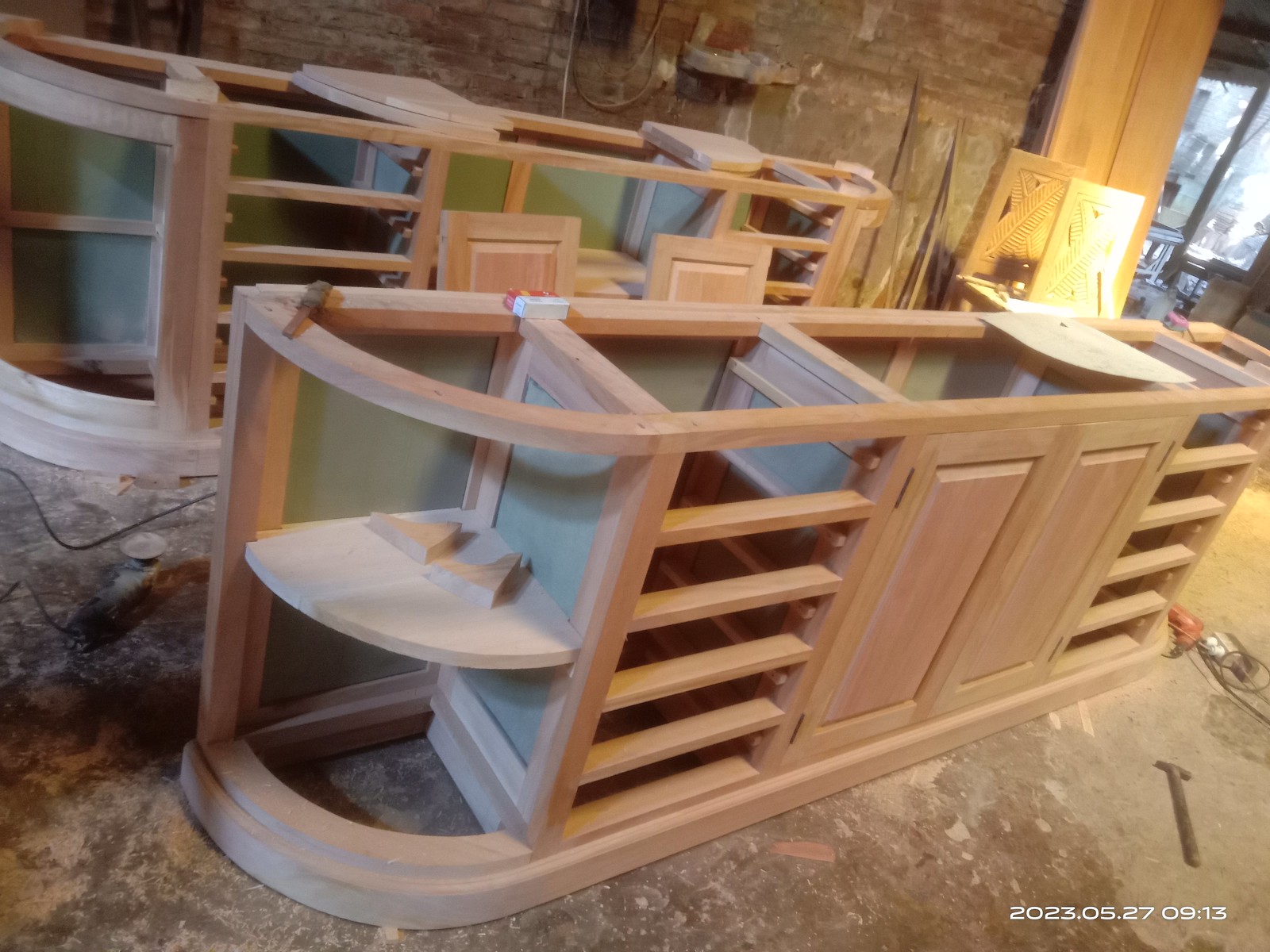The photograph captured indoors shows two sets of unfinished, light brown wooden cabinets positioned in a spacious workshop with a cement floor and an open layout. These cabinets, likely designed for a center island setup, lack countertops and have visible open frames. The shelves are partially built, with some rounded shelves on the far sides and no enclosed spaces yet. Among the shelves, several horizontal bars are noticeable. In the backdrop, an unfinished brick wall is highlighted with sunlight streaming through a window. A wooden shelf or cabinet is also present in the distance. A metal drill with a cord lies on the floor, adding to the work-in-progress atmosphere. The image has a timestamp in white lettering at the bottom that reads "2023-05-27-09-13".